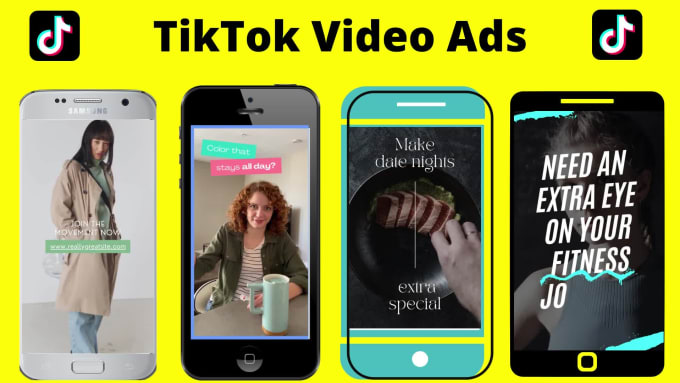The image is a desktop screenshot showcasing an advertisement for TikTok video ads against a vivid highlighter-yellow background. Centered at the top is the bold black text "TikTok Video Ads," flanked by the TikTok logo on both sides. The logo consists of a black square featuring a white musical note emblem.

Below the central text are four different smartphones arranged horizontally from left to right. These phones vary slightly in design, including differences in button placement and cutouts, suggesting a mix of older Samsung and Apple models. 

1. The phone on the far left is white and labeled "Samsung." It displays a video ad featuring a woman with long, straight brown hair wearing a white coat and blue jeans. The ad text reads, "Join the movement now," accompanied by a website URL that is too small to be legible.

2. The next phone presents a woman with reddish-brown curly hair wearing a black jacket and a black and white striped shirt. She is holding a tall green mug positioned on a gray countertop. The ad text states, "Stay fresh all day."

3. The third phone features an image of a hand holding a pan with meat, possibly being garnished. The ad text reads, "Make date nights extra special."

4. The final phone showcases an androgynous figure, potentially a white woman, dressed in a gray halter top. The accompanying text asks, "Need an extra eye on your fitness journey?"

Each phone displays a different potential TikTok video ad, illustrating various content styles and topics meant to engage users. Despite being shown on a desktop, the screenshot effectively captures the essence of mobile advertising on TikTok.